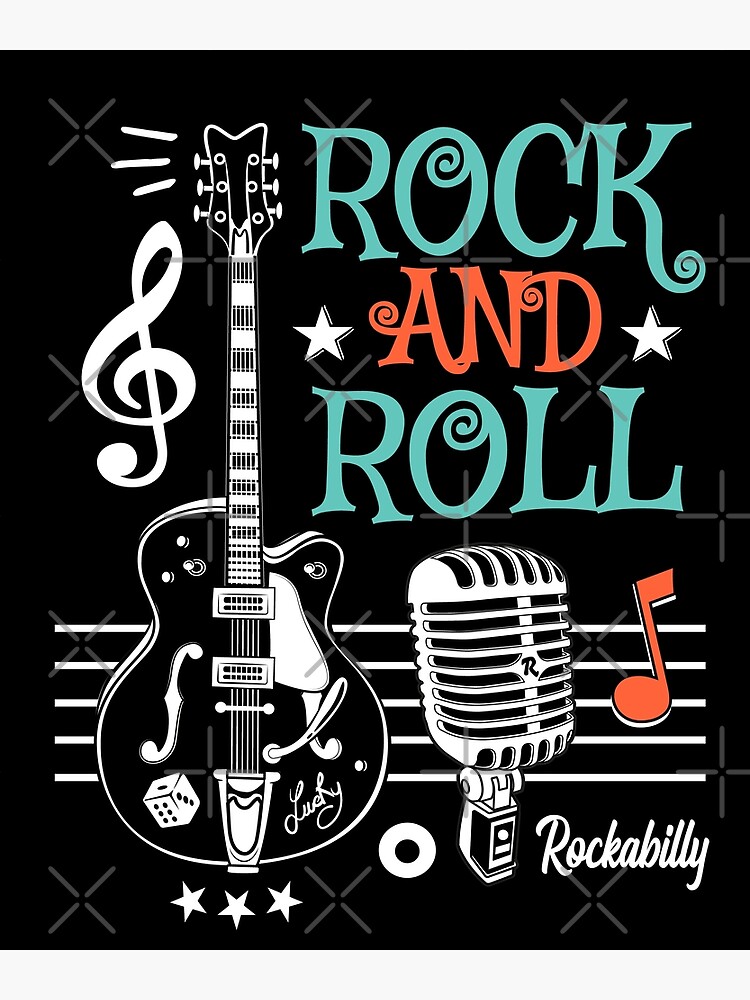This retro-style promotional poster features a striking black background adorned with crisp white musical staff lines that traverse the image. At the heart of the design, the bold words "Rock and Roll" take center stage, with "Rock" and "Roll" rendered in vibrant turquoise and the word "and" in vivid orange, flanked on both sides by white stars. An old-fashioned, black-and-white microphone with a steel grille, reminiscent of a classic car front, stands prominently on the lower right. Nearby, the word "Rockabilly," inscribed in elegant white cursive, anchors the corner. To the left of the microphone, a black electric guitar, reminiscent of a Fender, stands upright. The guitar is creatively adorned with a die, lending it an element of chance, and is labeled "Lucky" near its base. Scattered orange musical notes add a pop of color to this meticulously detailed composition. A delicate watermark comprised of repeating rows of gray axes and gray plus signs subtly decorates the background, enhancing the overall vintage aesthetic.